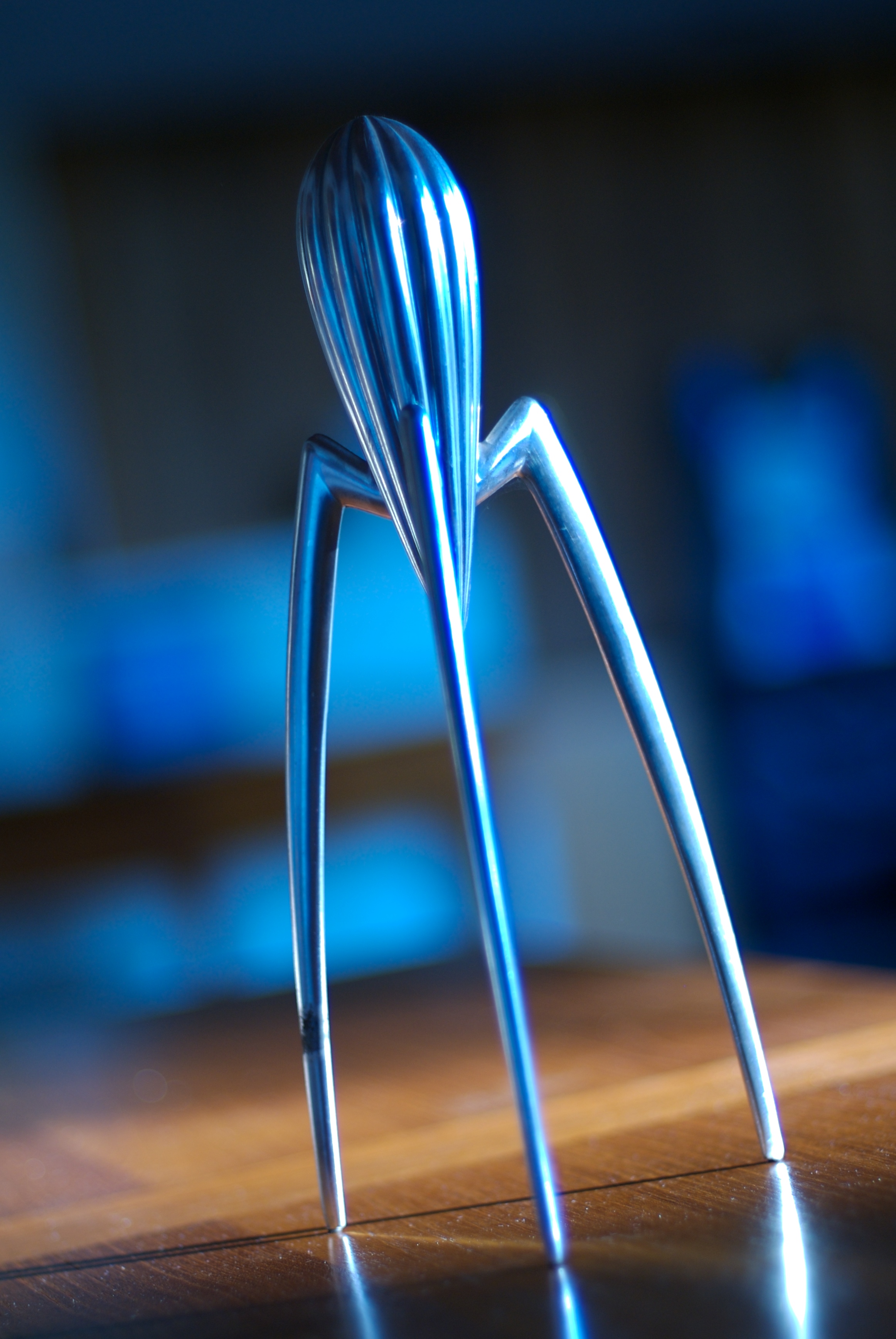In this close-up image, we see a peculiar metallic object set on a glossy brown wooden floor, which appears to be a table or desk. The surface exhibits different shades of brown. The object itself is strikingly reflective, catching the light from a source on the right side of the frame, making it shine brilliantly. The background is a blur of dark blues and blacks, ensuring all focus is on the object.

The structure resembles an elongated, narrow 'M', with three long legs similar to a tripod's, spaced out equidistantly, supporting it. The legs are approximately two to three inches long each. At the top of the legs sits a narrow, bulbous shape, akin to a hot air balloon, complete with vertical grooves running down its metallic surface. This upper part measures about an inch to an inch and a half in height. Its reflective blue metal sheen adds an element of intrigue, suggesting an abstract or potentially alien design. The object is tilted slightly to the left, adding to its whimsical and enigmatic appearance.